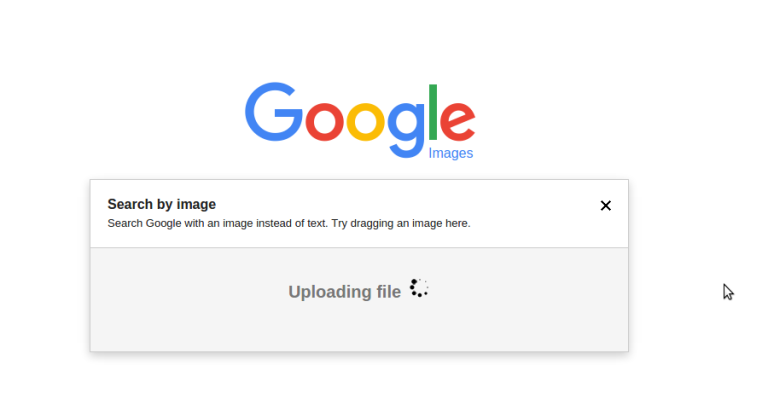The image is a screenshot from Google Images with a clean, white background. Centered at the top is the iconic Google logo, featuring the word "Google" in various colors: the 'G' is in blue, the 'o' is red, the second 'o' is yellow, the lowercase 'g' is also blue, the 'l' is green, and the lowercase 'e' is red. Directly below the logo, in a smaller blue font, is the word "Images."

Beneath the title, there is a large, outlined box divided into two sections. The outline of the box is gray. The top section of the box contains the text "Search by Image" in a bold black font. Just below this, in a smaller, italicized font, it reads, "Search Google with an image instead of text. Try dragging an image here." On the top left corner of this section is a black 'X' icon.

The bottom section of the outlined box displays the text "Uploading file..." in a gray font that matches the size of the "Search by Image" text above. Below this text, there is an animation of little dots forming a circle, indicating the progress of the file upload. The dots on the left side of this circle are black, showing that the upload is in progress, while the remaining dots are gray. On the far right side, outside of the outlined box, there is a white mouse pointer.